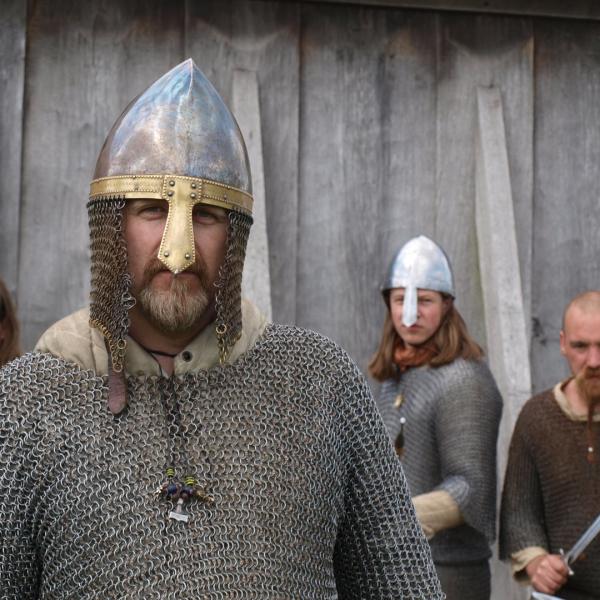The photograph depicts three individuals clad in medieval-style armor, evoking a Viking-era theme reminiscent of "Monty Python and the Holy Grail." The person in the foreground, positioned to the left, is prominently featured wearing chainmail armor over a tan garment. His shiny, dome-shaped metal helmet adorned with a gold band and a protective nose guard further enhances his imposing presence. The helmet also includes a chainmail drape that extends around the sides and back of his head. He bears a beard and wears a long necklace with an emblem or weapon, adding to his authentic appearance. 

Behind him, on the right side of the image, stand two other individuals dressed similarly in chainmail armor. One is partially visible, donned in brown chainmail, and brandishing a sword, sporting a beard and mustache. The other, situated closer to the wooden, grayish-light brown wall in the background, wears all-silver armor, featuring a matching silver dome-shaped helmet with a distinctive nose guard. This individual also has facial hair akin to the one in the foreground. The wooden building in the backdrop subtly frames the scene, enhancing the historic ambiance.